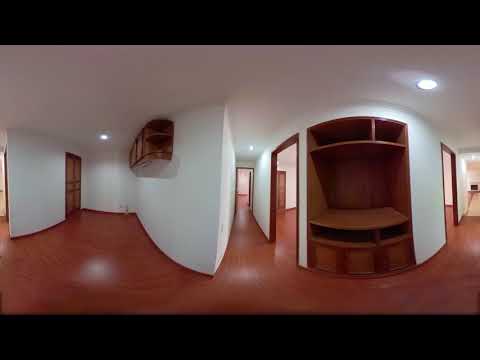The image depicts the interior of a vacant house captured with a fish-eye lens, resulting in a noticeably warped perspective where the central walls curve inward, creating a circular effect. The flooring appears to be a reddish-brown plank, albeit slightly blurry, which may indicate that the photo was taken with an older camera. The white ceilings and walls are uniformly illuminated by white pot lights. Prominently centered within the image is a built-in brown shelf within the main white wall. This shelf includes a large open space in the middle, possibly designed for an entertainment center, flanked by shelving on the top and bottom, and cabinets at the base. To the left of the image, there's a brown closet door and what appears to be a kitchen area, identified by wooden cabinets installed high on the wall, likely close to the ceiling. On the right side of the hallway, another doorway is visible, suggesting access to possibly a bedroom. The hallway extends into the background, ending at another doorway, enforcing the emptiness and depth of the scene. The wood accents throughout the space, from the kitchen cabinets to the framing around the doors, maintain a consistent brown tone, enhancing the house's cohesive yet deserted appearance.